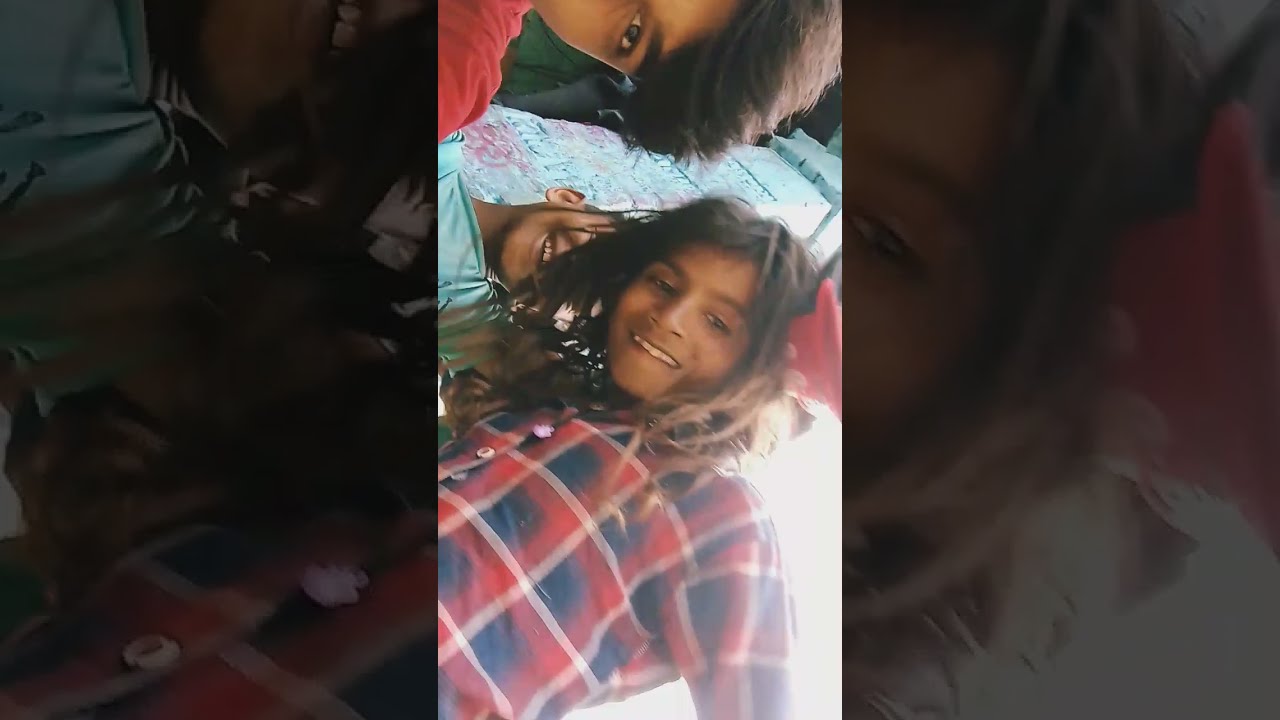This vibrant, daytime exterior photograph captures a joyful moment among three children of South American or Indian ancestry, their warm-hued skin radiating in the natural light. The image, slightly rotated, centers on a young girl with long, dark, somewhat messy hair, wearing a red, white, and blue plaid flannel shirt. Her broad smile, dark eyes, and showing teeth convey happiness and friendliness. Behind her, a boy in an aqua shirt peeks through, his short dark hair and cheerful expression contributing to the lively scene. At the top of the image, somewhat obscured, is another boy with short, stylishly brushed hair, wearing a red shirt. The photograph's unusual angle accentuates their playful spirits, with the actual photo in the center and a blurred, darkened background adding depth, while a blue stone pillar subtly grounds the image. Each child’s smile and casual attire underscore their cheerful, carefree demeanor, making the moment feel spontaneous and full of fun.